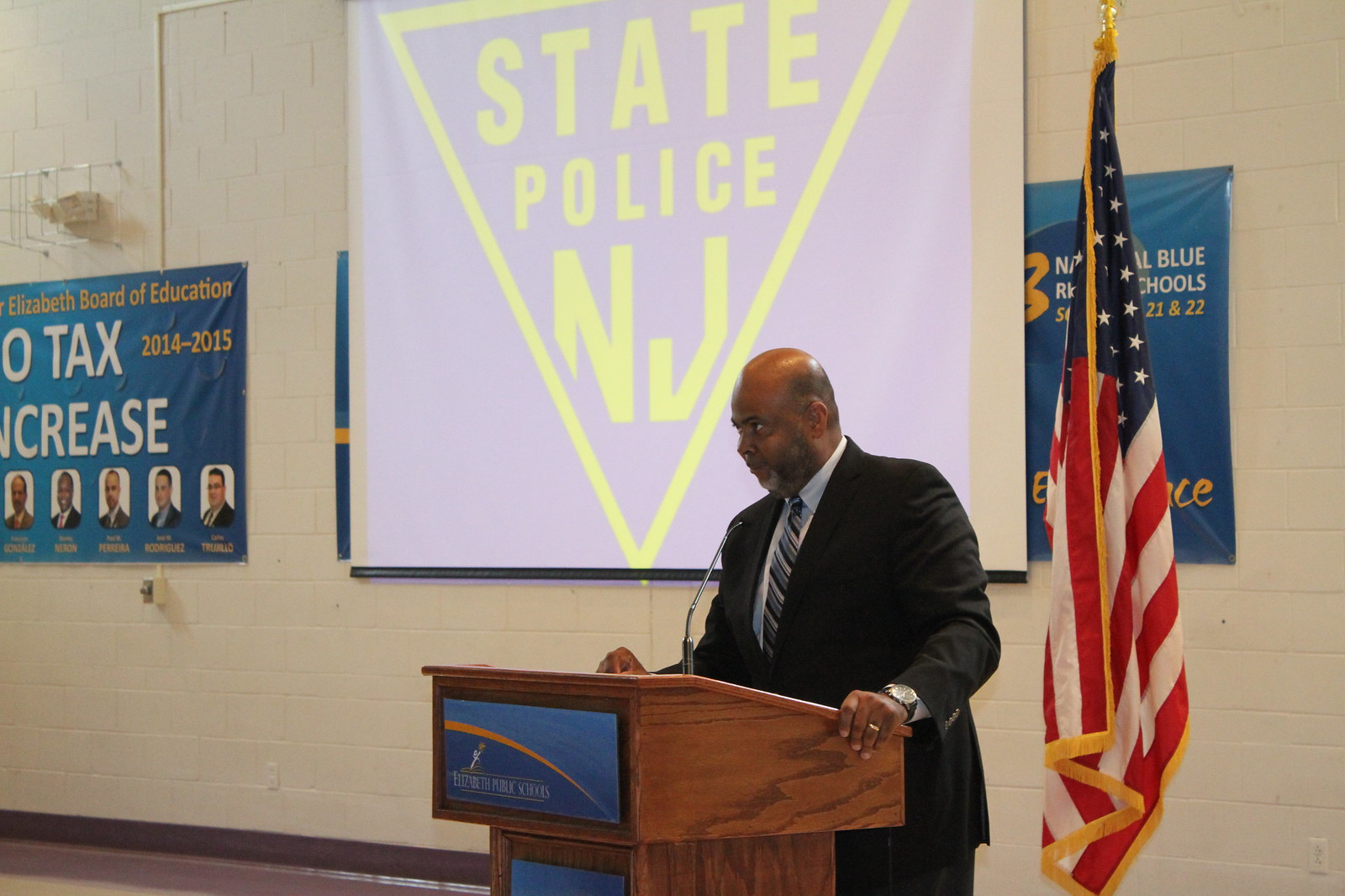This photograph captures a man of Indian descent, dressed in a black suit with a gray, black, and white striped tie, standing at a light brown wooden podium adorned with a blue plaque that reads "Elizabeth Public Schools." He appears to be giving a speech, talking into a microphone positioned on top of the podium. An American flag on a pole stands to his right. Behind him, a projection screen displays an image with a blue background and an upside-down yellow triangle containing the words "State Police NJ." The setting seems to be an auditorium with white walls adorned with various banners, including blue ones with white writing and photos.